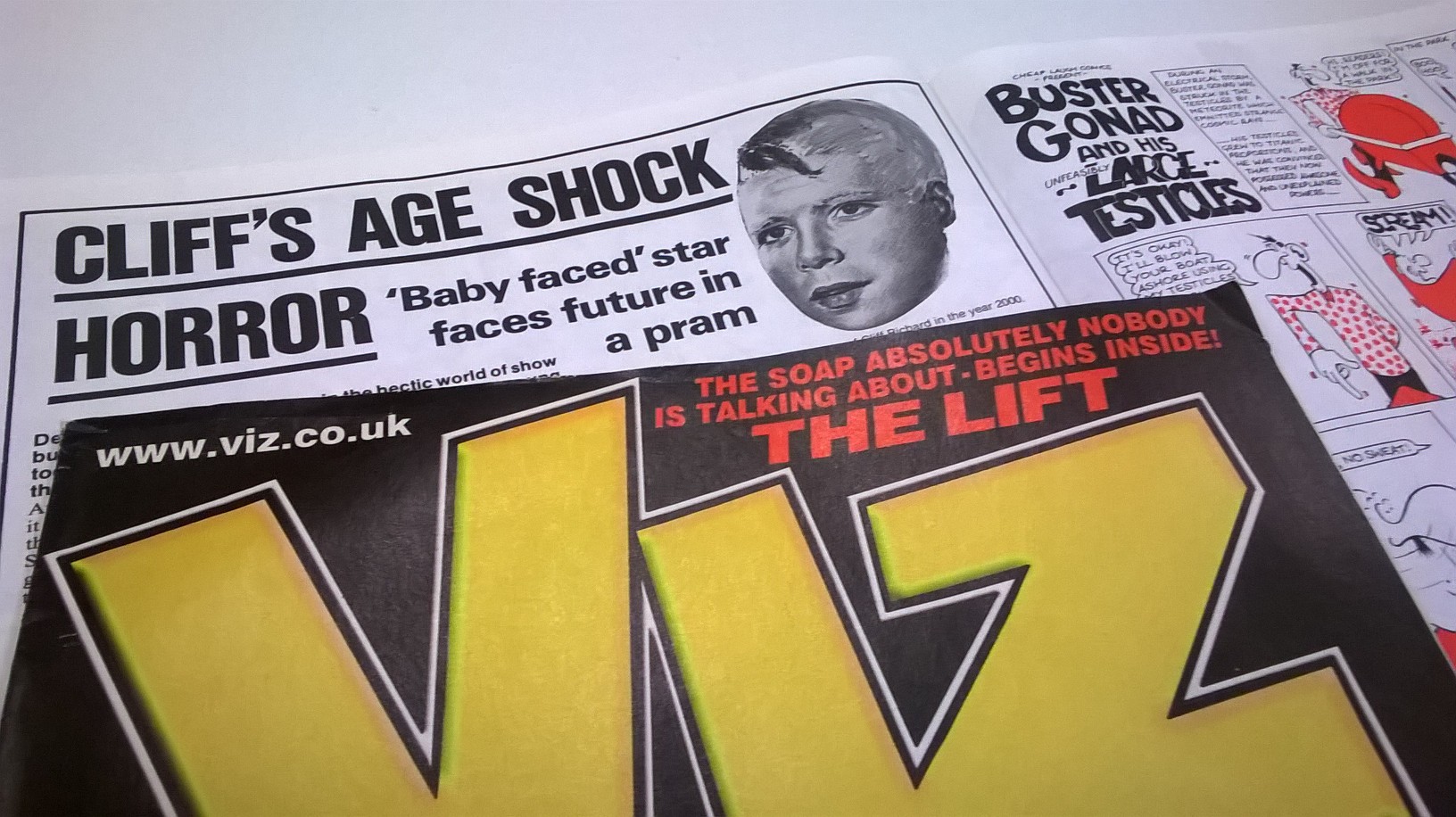In this landscape-oriented photograph, a close-up shot reveals a magazine open in the middle, lying on a white table, with an additional black magazine insert perched on top. The magazine insert prominently displays the letters "VIZ" in bold yellow font, centered on a black background with a white outline around the letters. The top left corner of this insert includes the URL "www.viz.co.uk" in white font, while the top right corner features the text "The Soap Absolutely Nobody Is Talking About Begins Inside The Lift" in striking red font. Beneath this insert, the visible pages of the opened magazine have a clean, white background with an assortment of black, red, and yellow text. The left page reads "Cliff's Age Shock Horror, Baby Face Star Faces Future in Pram" alongside a stylized illustration of a human face looking to the left, possibly depicting a "young boy." The colors throughout include a blend of white, black, red, and yellow, and the composition is dominated by the juxtaposition of the two magazines, one stacked atop the other, creating a visually dynamic and layered effect. The setup appears to be a casual arrangement on a table, with the main elements clearly in focus and positioned largely in the center of the image.